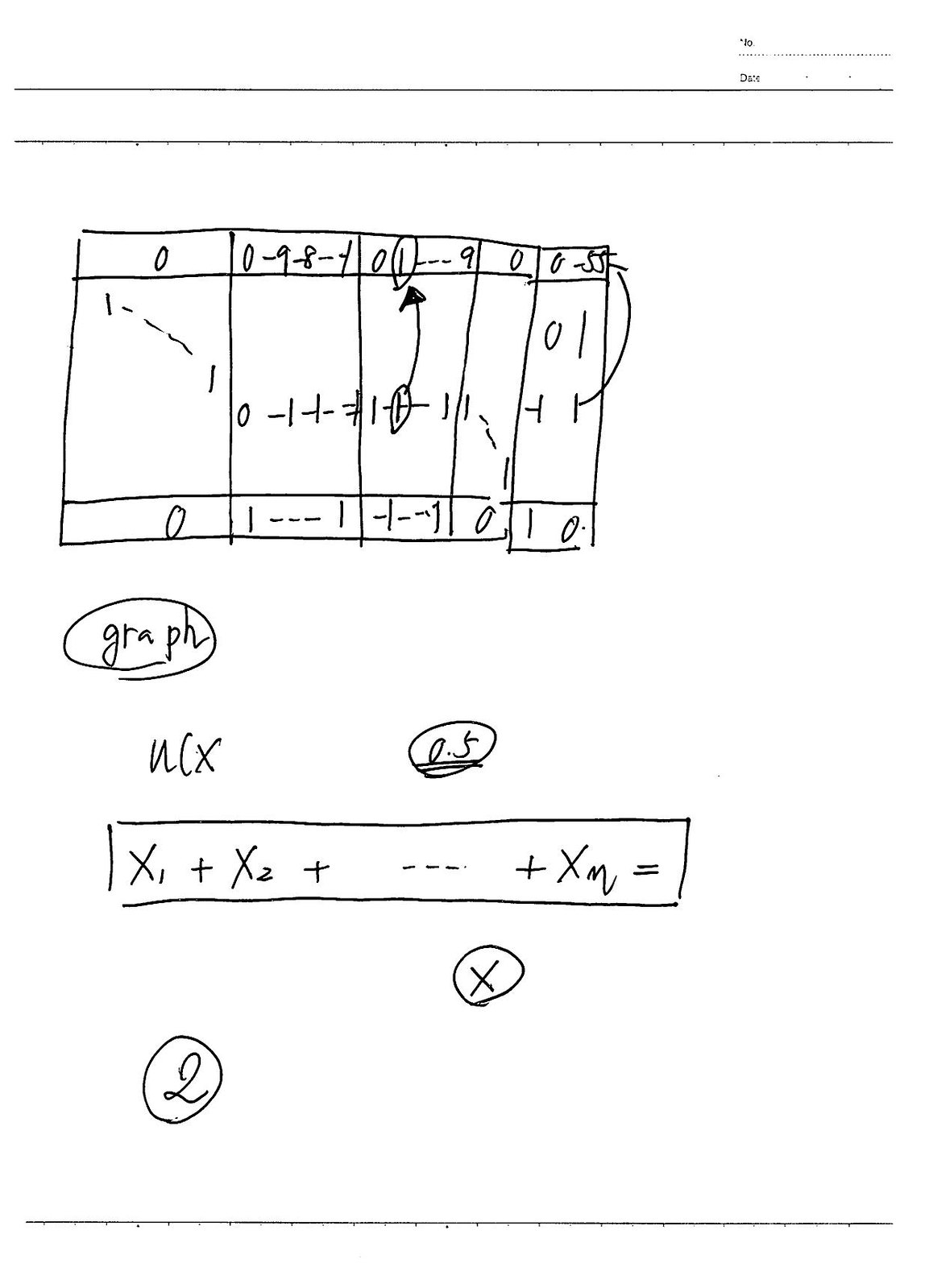This image appears to be a handwritten sketch done on a table. In the upper left corner, there is a table that consists of three rows and four columns. 

- **First Row:** 
  - First cell: "0"
  - Second cell: "0"
  - Third cell: "-9 -8 -1"
  - Fourth cell: "0 (1) - - - 9"
  - Fifth cell: "0"
  - Sixth cell: "0"
  - Seventh cell: "-5"

- **Second Row (a taller/wider row):**
  - First cell: "1 ---"
  - Second cell (diagonal entry): "1"
  - Third cell: "0 -1 -1 -1"
  - Fourth cell: "0 (1) --- 1"
  - Fifth cell: "0"
  - Sixth cell: "1 - 1 0" (with a line sweeping up to the top of the column)

- **Final Row:**
  - First cell: "0 (1) --- 1"
  - Second cell: "1 - 1"
  - Third cell: "0 1"
  - Fourth cell: "1"
  - Fifth cell: "1 (below)"
  - The word "graph" is circled beneath this row.

Additionally, there is an equation enclosed in rectangular boxes below the table:
- "X₁ + X₂ + --- + Xₘ ="

  Below this equation:
  - To the left: "2" (circled)
  - To the right of the center: "X" (circled)

These seem to be notes where someone is attempting to solve an equation or problem. All writing is handwritten in black pen, and no other text or print is visible.